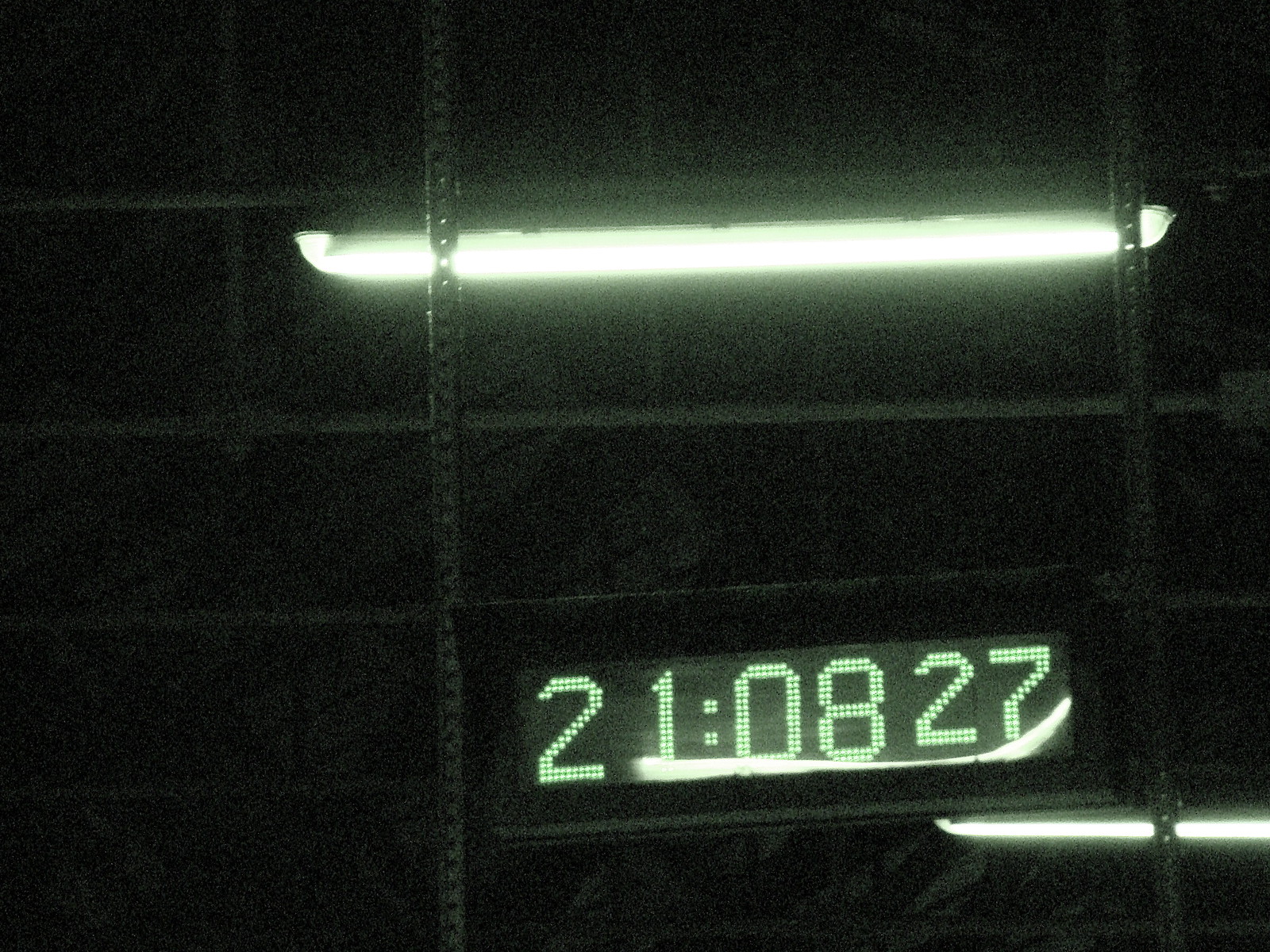The image showcases a sleek black shelving unit adorned with vibrant neon lighting. On the second shelf, a vivid green neon light stretches across, casting an ethereal glow on the surrounding surfaces. Just below, on the third shelf, a digital display clock prominently reads "21:08:27" in bright digits. A reflection or possibly another hidden neon light can be seen below the clock, adding to the layered illumination effect. The overall scene is bathed in contrasting neon hues, giving the shelves a futuristic and visually captivating appearance.